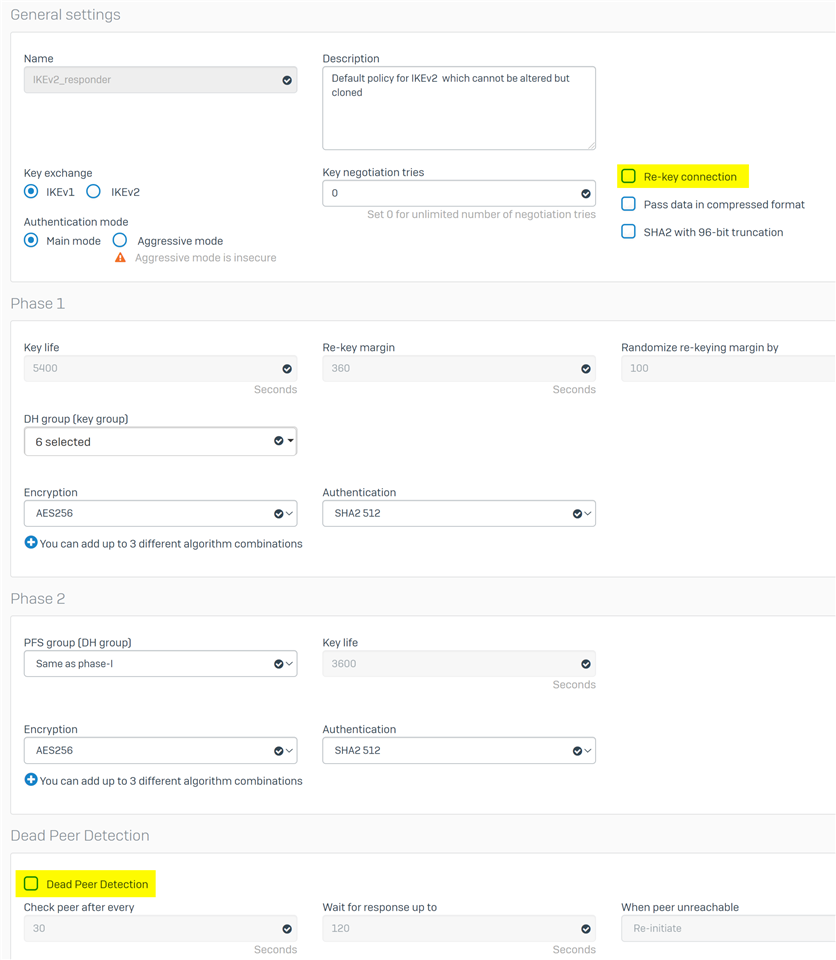This image depicts a settings menu for a web-based service with a clean, white background. In the top left corner, there is a heading labeled "General Settings," indicating that this section pertains to the general configurations of the service. At the top of the menu, there are fields for "Name" and "Description," followed by numerous advanced settings.

One section, highlighted in yellow, is labeled "Rekey Connection." Below this, Phase 1 settings include fields for "Key Life," "Rekey Margin," "Randomized Rekey Margin by," "DH Group," "Encryption," and "Authentication." Moving down, Phase 2 settings are detailed with options for "PFS Group," "Key Life," "Encryption," and "Authentication."

The final section is titled "Dead Peer Detection," featuring a highlighted yellow option within a checkbox. The settings specify to "Check Peer After Every (specified interval) for a response" and actions for "When Peer Unreachable." This comprehensive settings menu allows for detailed customization and management of the service's various security and operational parameters.